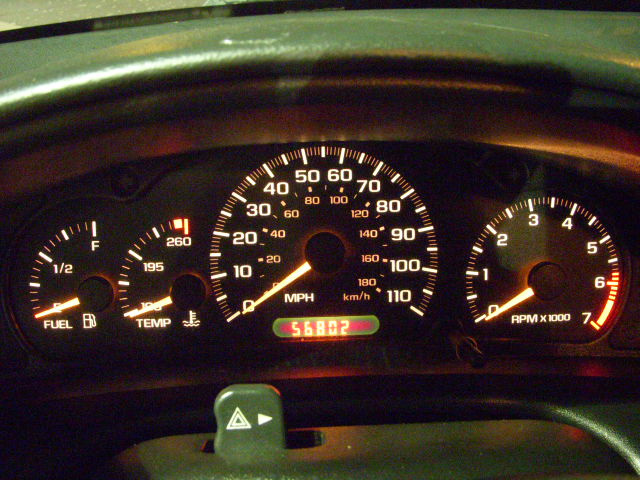This detailed photograph captures the dashboard of a car, showcasing four illuminated analog dials that provide various vital readings for the driver. At the center of the image, the prominent speedometer is feature, marked in both miles per hour (ranging from 0 to 110) and kilometers per hour (ranging from 0 to 180), with clear numbers and backlit pointers enhancing visibility. To the right of the speedometer is a slightly smaller dial reading RPM (Revolutions Per Minute), scaled from 0 to 7 (or 7,000 RPM). On the left, there are two half-sized dials; one indicates the engine temperature up to 260 degrees, and the other displays the fuel level, from empty to full, with a clear midway point. At the bottom of the dashboard, a noticeable button marked with a triangle and an arrow can be seen, which is used for activating the car's four-way flasher signals. Each element is detailed, backlit, and designed for clear and precise readings, contributing to the functionality and safety of the vehicle.